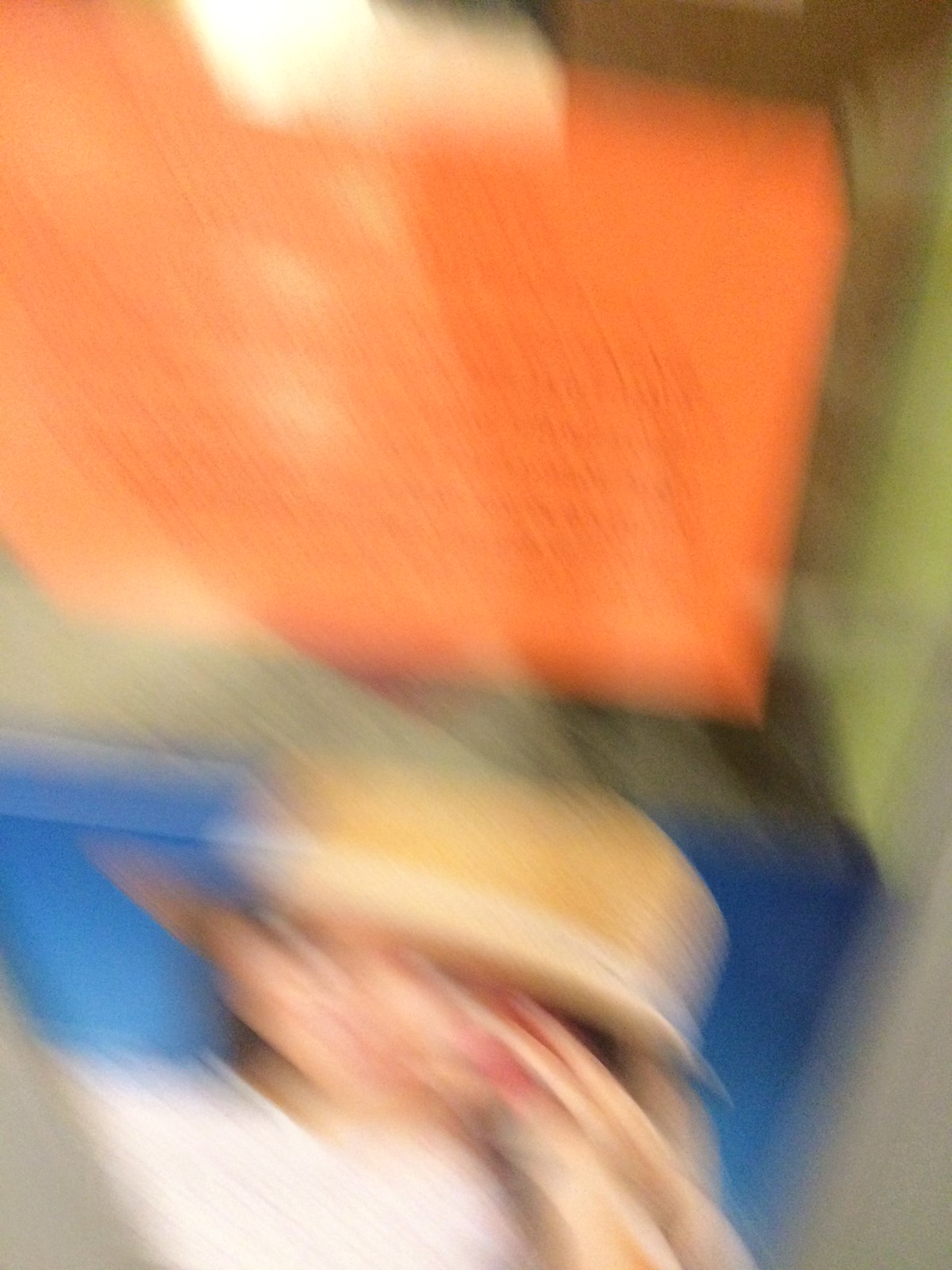This is a detailed description of a very blurry image. At the top of the image, there is an orange rectangular object, the nature of which is unclear - it could be a box or a suitcase. Below this rectangle, there's a picture of a woman set against a blue background. The woman appears to be wearing a small, close-fitting straw hat that doesn't flare out much. She has blonde hair and possibly brown eyes, and she seems to be looking to the right. Her hand, which is also blurry, looks like it might be touching her eye. She appears to be wearing a white v-neck shirt.